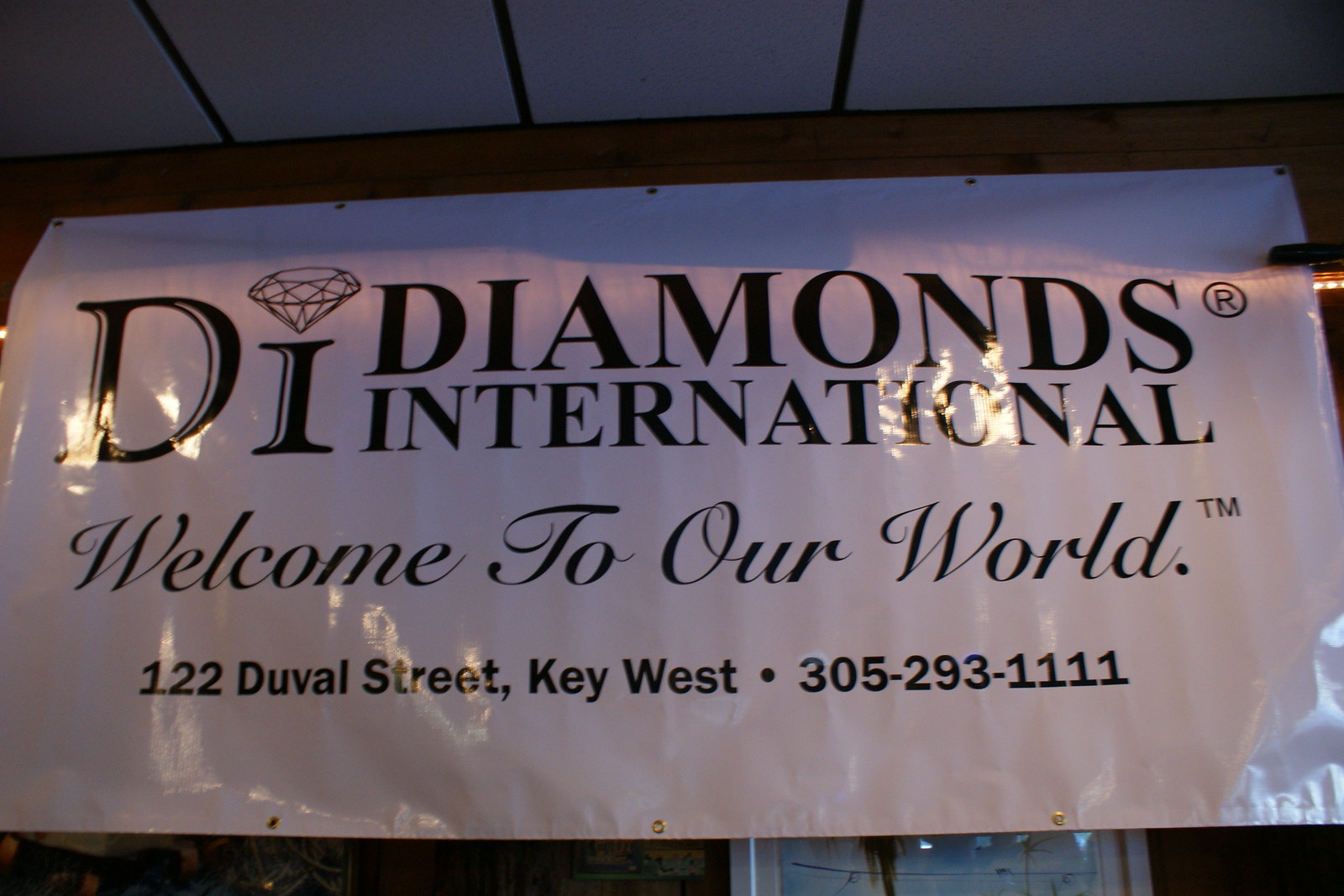The photograph depicts a large white plastic sign, resembling a tarp, securely fastened to a wall with metal rivets at the top and bottom. The sign's text is printed in clear, black letters. At the top, "DI" is prominently displayed with an image of a diamond above the "I". Below this, "Diamonds International" is written, followed by the script phrase "Welcome to Our World." Towards the bottom of the sign, the address "122 Duval Street, Key West" is listed, accompanied by the phone number "305-293-1111." The sign's clean and bright appearance is highlighted by the natural light in the setting.